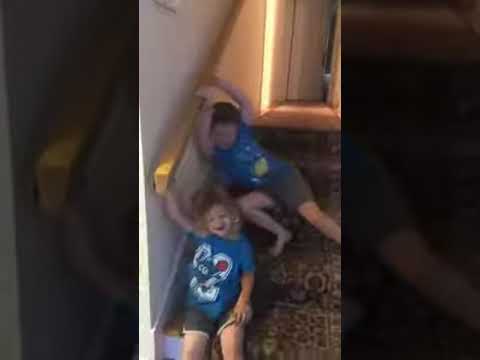In this grainy, low-quality image, we observe a small, carpeted staircase situated indoors, likely within a residence. The focal point is two young children sitting on the stairs, both clad in blue shirts adorned with designs. The child at the bottom of the stairs has short blonde hair, with her right hand resting against the wall, while the child above her, with short brown hair, sits a step higher, grasping the wooden handrail on the left with both hands. At the top of the staircase, there's a hallway with a couple of open doorways visible, allowing light to filter through. The staircase carpet features dark tones with intricate patterns, contrasting the light-colored surrounding walls and the yellow handrail on the left side. The overall scene appears slightly dark and the image quality is poor, contributing to the graininess and difficulty in discerning finer details.